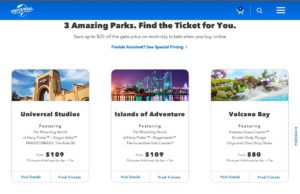The image depicts a web page showcasing multiple travel options from Universal Pictures. The top of the page is highlighted by a blue navigation bar featuring the white Universal Pictures logo on the left. On the right side of the bar, there's a white shopping cart icon with a dark blue circle containing the number "1." Adjacent to it is a white separator line, followed by a white magnifying glass icon, and then three horizontal white lines representing a menu.

Beneath the navigation bar, the background changes to white. At the top in black text, it reads: "Three Amazing Parks, Find the Ticket for You." Below this header, there's some gray text which is illegible due to low resolution, accompanied by illegible blue text with a right-pointing arrow.

The main content area is divided into three sections, each representing a different park option:

1. **Universal Studios:** The first option features an image of a studio entrance framed by a beige arch and surrounding walls, set against a blue sky with white clouds. Below the image, there's some illegible gray text followed by the price in black text: "$109."

2. **Islands of Adventure:** The second option shows a nighttime scene of a roller coaster or similar amusement ride. This section also includes illegible gray text and lists the price: "$109."

3. **Volcano Bay:** The final option displays a picture of a theme park featuring a beach area, blue water, green foliage, and a clear blue sky. The listed price for this attraction is: "$80."

These detailed descriptions of each park option provide users with a visual and textual overview to help them make an informed decision.